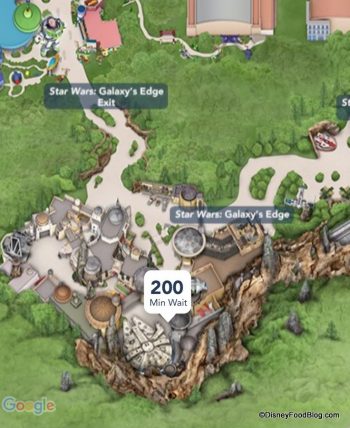The image features a detailed, colorful map that highlights various geographical and structural elements. On the upper left side, there's a partial blue circle with a green circle on top of it, possibly indicating a water body or a landmark. The map displays areas abundant with grass, interspersed with buildings that are predominantly tan, terracotta, and gray. Roads and trees are also depicted across the map, adding to its detailed layout.

In the upper portion of the map, there is a semi-transparent gray rectangle with the text "Star Wars: Galaxy's Edge Exit." Another similar rectangle, further down and towards the right, reads "Star Wars: Galaxy's Edge." Towards the lower part of the image, there's a white shape resembling a square with rounded corners and a triangular point at the bottom, inside which it states "200 m.” At the bottom left corner, the familiar multicolored "Google" logo is visible. Additionally, there are some symbols and text on the right side of the map, although they're not easily discernible.